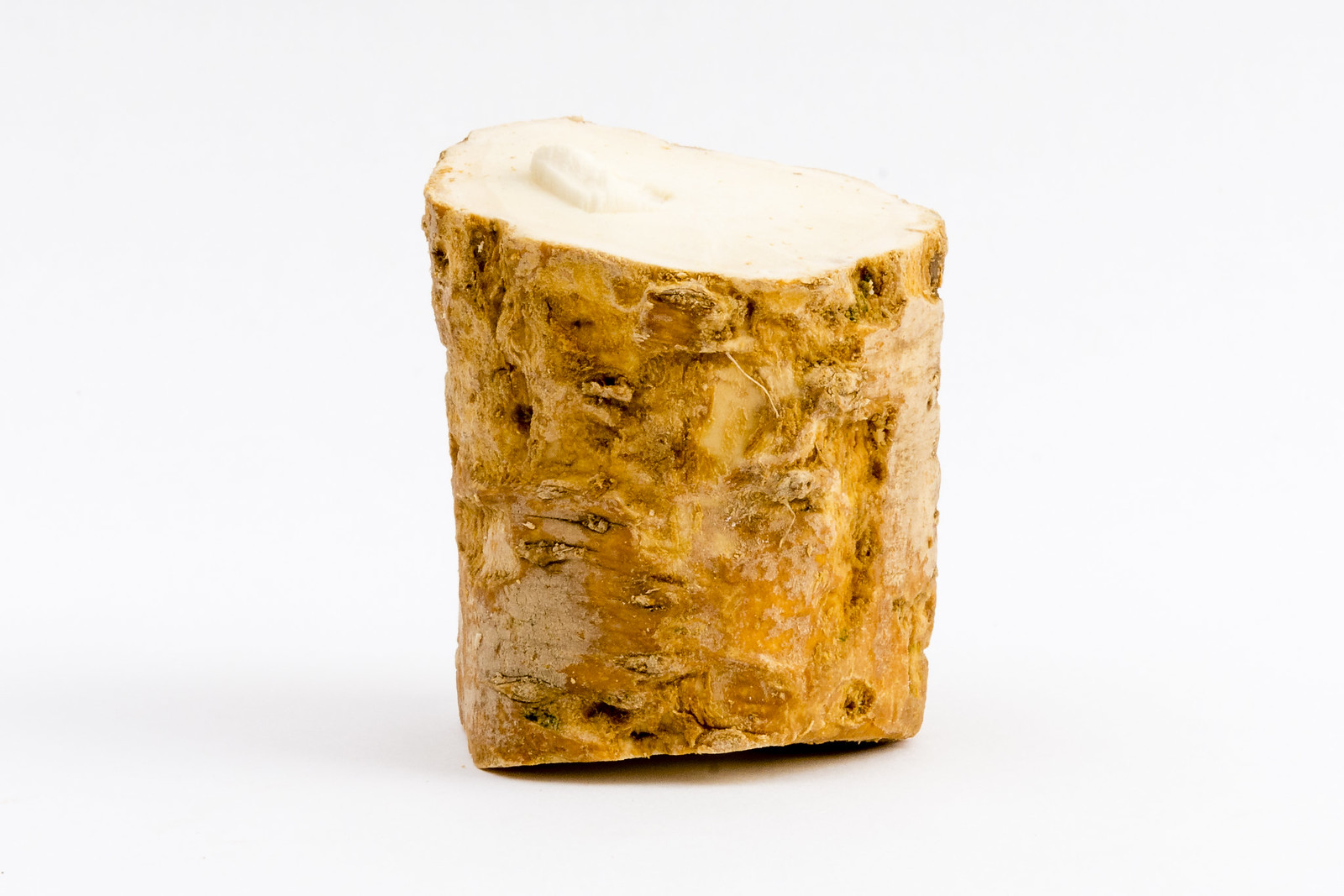A detailed photograph depicts a central cylindrical object that appears to be a wooden log or possibly petrified wood, set against a stark white, empty background. The log stands approximately a couple of feet tall, displaying a mottled surface with various shades of brown, ranging from light brown to darker amber tones. The outer edge of the log is rugged and scraped, suggesting a rough, uneven texture. The top of the log is notably lighter, almost white, possibly due to the reflection of light, with a conspicuous white splash or dollop enhancing its bright appearance. The object casts a shadow below, accentuating its uneven bottom and hinting at its considerable weight.